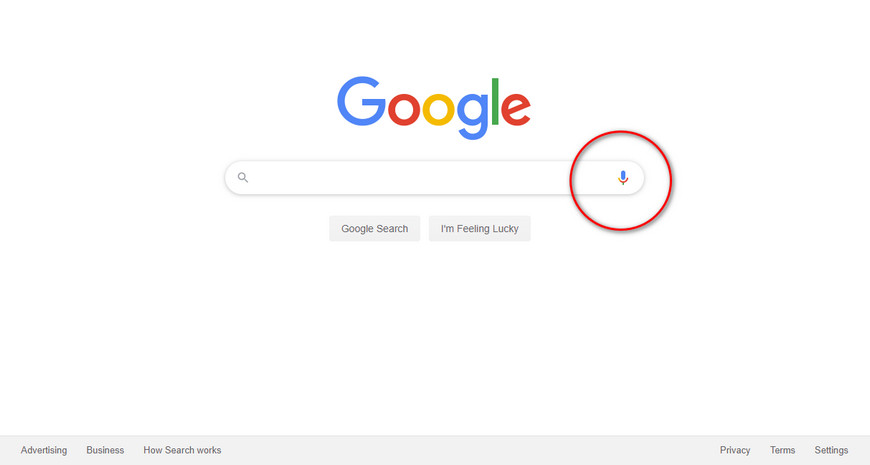The image is a screenshot of the Google homepage, presented in a landscape orientation, roughly one and a half to two times wider than it is tall. The background is predominantly white, blending seamlessly into the surrounding margins, which adds to the minimalist and clean design.

At the top center of the image, the large and colorful Google logo is prominently displayed. Below the logo is the classic horizontal search bar, featuring a gray magnifying glass icon on the left side. The search bar itself has a rounded rectangle shape. On the right edge of the search bar is a microphone icon, colored blue at the top and red at the bottom, which is circled in red, emphasizing its importance or the intention to draw attention to it.

Directly beneath the search bar are two buttons: the left button reads "Google Search" and the right button reads "I'm Feeling Lucky," both in black text and set atop light gray, rounded rectangular buttons.

At the very bottom of the image is the footer, divided into two sections. To the left, it displays links for “Advertising,” “Business,” and “How Search Works.” To the right, it features “Privacy,” “Terms,” and “Settings.” The overall layout and subtle highlighting serve as an illustrative representation of the typical, user-friendly Google homepage.